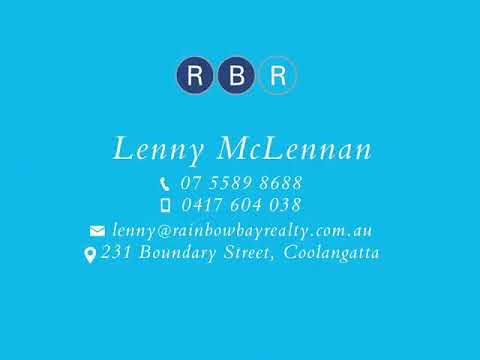A digital business card for Lenny McLennan features a medium blue background with an emblem comprising three circles at the top center. The first circle on the left is dark blue with a white 'R', the circle in the middle is the same dark blue with a white 'B', and the circle on the right is light blue, matching the background, with a white 'R', spelling out 'RBR'. Below this emblem, in white text, is the name Lenny McLennan. Beneath the name, there is a phone icon followed by the number 07-5589-8688. Below this, there is an icon resembling a smartphone with a number: 047-0417-604-038. Following this is an email icon with the address Lenny@rainbowrealty.com.au, and at the bottom, a location pin icon with the address: 231 Boundary Street, Kulangara.